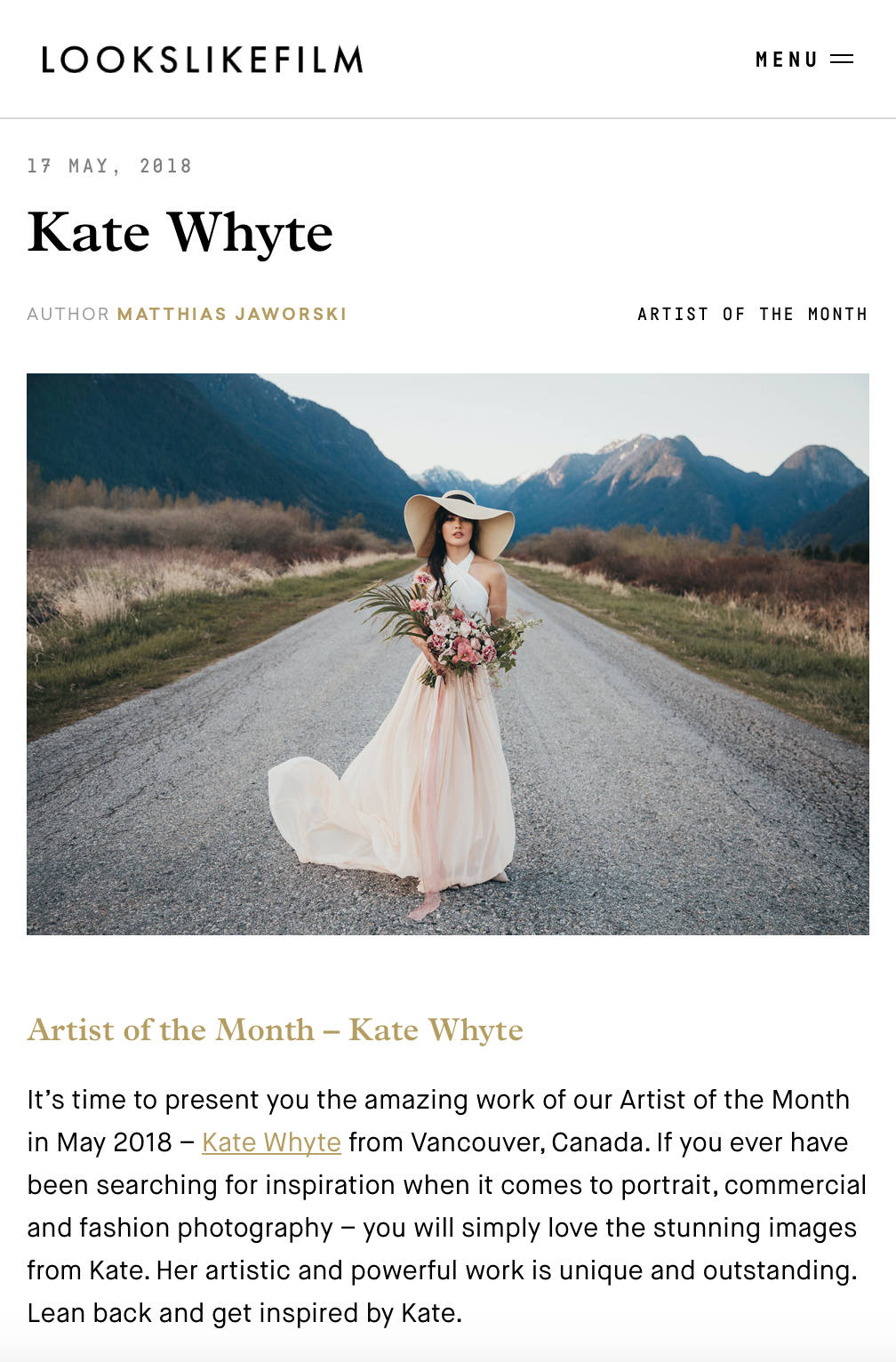The screenshot captures a mobile webpage featuring a bold header displaying the word "FILM" in all uppercase letters. On the right side of the header, there is a menu button labeled "EU" in uppercase text, accompanied by two horizontal bars in a single row. Just below the header, a thin gray line extends across the screen from left to right.

Below the line, the date "17 May, 2018" is displayed, followed by the name "Kate Whyte" in black text, which is slightly larger than the surrounding text. Underneath, the author "Matthias Jaworski" is highlighted in yellow.

On the right side of the screen, a section titled "ARTISTS OF THE MONTH" is prominently displayed in all capital letters. An image follows, depicting a woman in a flowing dress, which could be either a sundress or a wedding dress. She is wearing a large hat that covers her head and shoulders. In her hands, she holds a bouquet of mixed flowers, possibly carnations.

Below the image, another caption reads "ARTISTS OF THE MONTH - K. WHITE," followed by a detailed description of Kate Whyte, including information about her background and other relevant details.